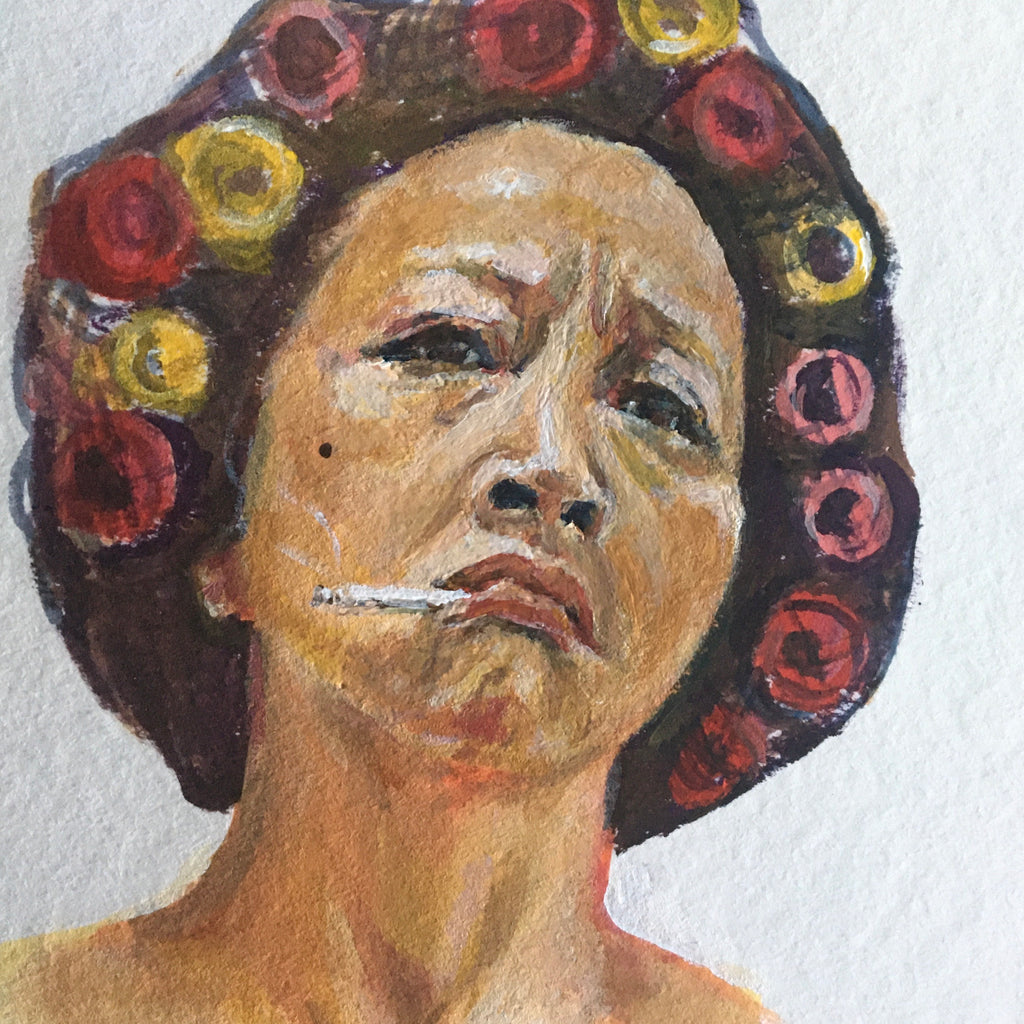The painting depicts a woman, possibly of Asian or Filipino descent, facing the viewer on an off-white to gray background. She appears haggard and weathered, likely in her mid-forties, with tired, defeated eyes and scowling marks between her eyebrows. Her lips are puckered in a scowl, accentuated by the red lipstick she wears, and from the right side of her mouth dangles a cigarette, with visible ash and a wisp of smoke curling up beside her face. Her hair, a dark brown color, is encircled by an assortment of hair rollers in red, pink, and yellow hues, all held in place by a hairnet. The detailed depiction suggests that she might be either preparing for the day or unwinding after a long day, embodying a sense of fatigue and solemnity.